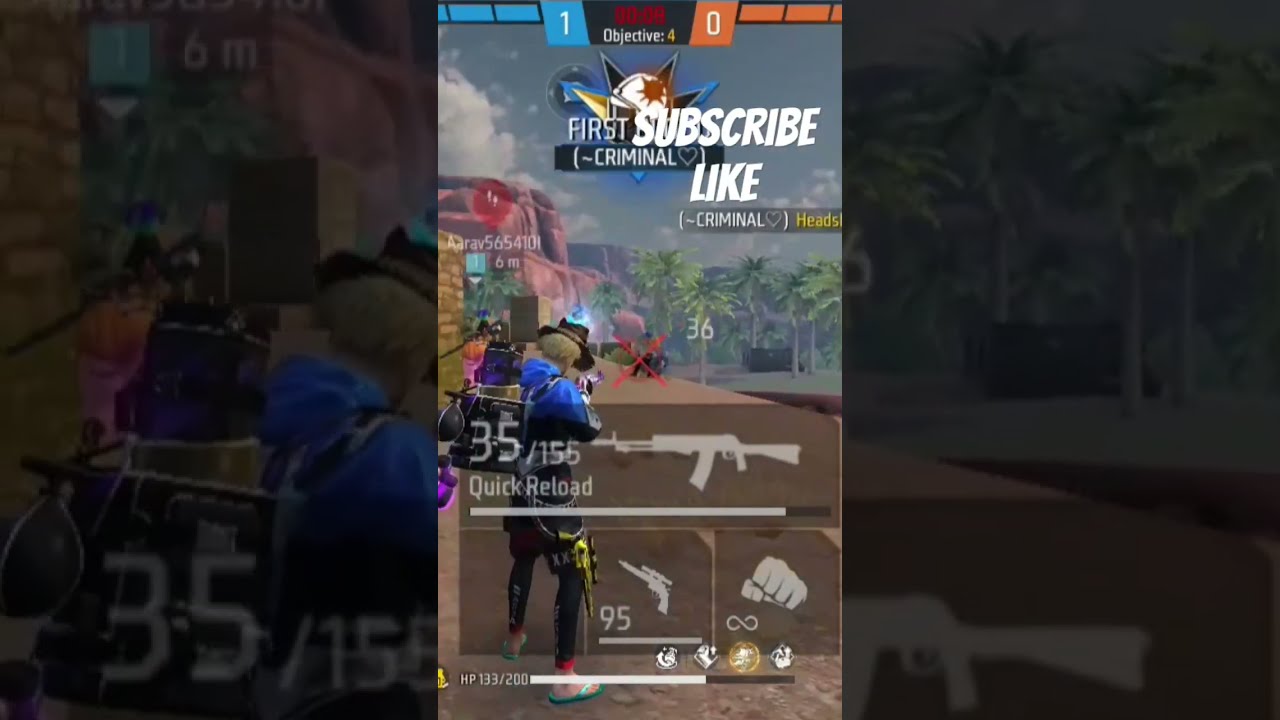In this image, we see a screenshot from a video game, possibly captured from a TikTok or Instagram live stream due to its portrait orientation and multiple rectangular boxes on the sides. The focal point is a character standing near the bottom left of the screen, engaging in combat. The character wears a blue jacket, pants, a cowboy hat, flip-flops, and a backpack, and wields a gold sniper rifle hanging from their leg and a purple gun in hand. They're shooting at an opponent in the distance, marked by a red X.

The interface includes various elements: at the very top, there is text in white reading "subscribe and like," indicating the image may be from a streaming platform. The top section also features a score with a blue bar on the left marked "1" and an orange bar on the right marked "0," alongside a clock displaying "Objective 4" with eight seconds remaining.

The bottom of the screen displays a menu for quick reloads and swapping between different guns, suggesting options for both ranged and hand-to-hand combat. The overall setting is dimly lit and somewhat dark, yet the environment is vividly colored with an array of light blue, red, black, blue, purple, pink, brown, gray, and green hues. No single element is centered, adding to the scattered and dynamic feel of the image, emphasizing the chaotic and fast-paced nature of the gameplay.